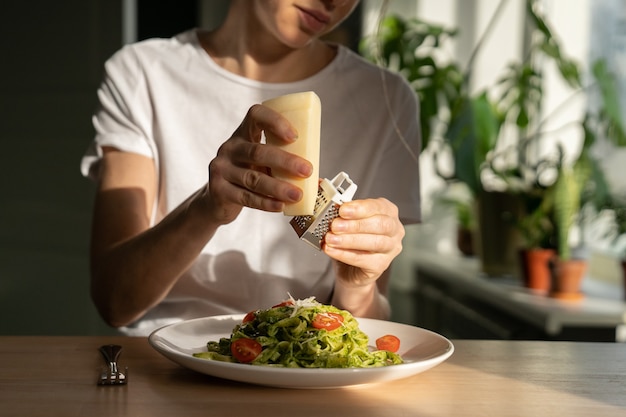In this image, a woman with short hair, dressed in a plain white t-shirt, is seated at a wooden mahogany table. She is diligently grating a large block of cheese with a small cheese grater, adding the freshly shredded cheese to her salad. The salad, which includes sliced tomatoes and a clear dressing, perhaps oil-based, is presented on a white porcelain dish. Nearby, a fork rests on the bottom left side of the plate. The table is bathed in sunlight, reflected off the table and her shirt, indicating that it is a sunny day. In the blurred background, several houseplants are visible, positioned on a windowsill or shelf, adding a touch of greenery to the scene.